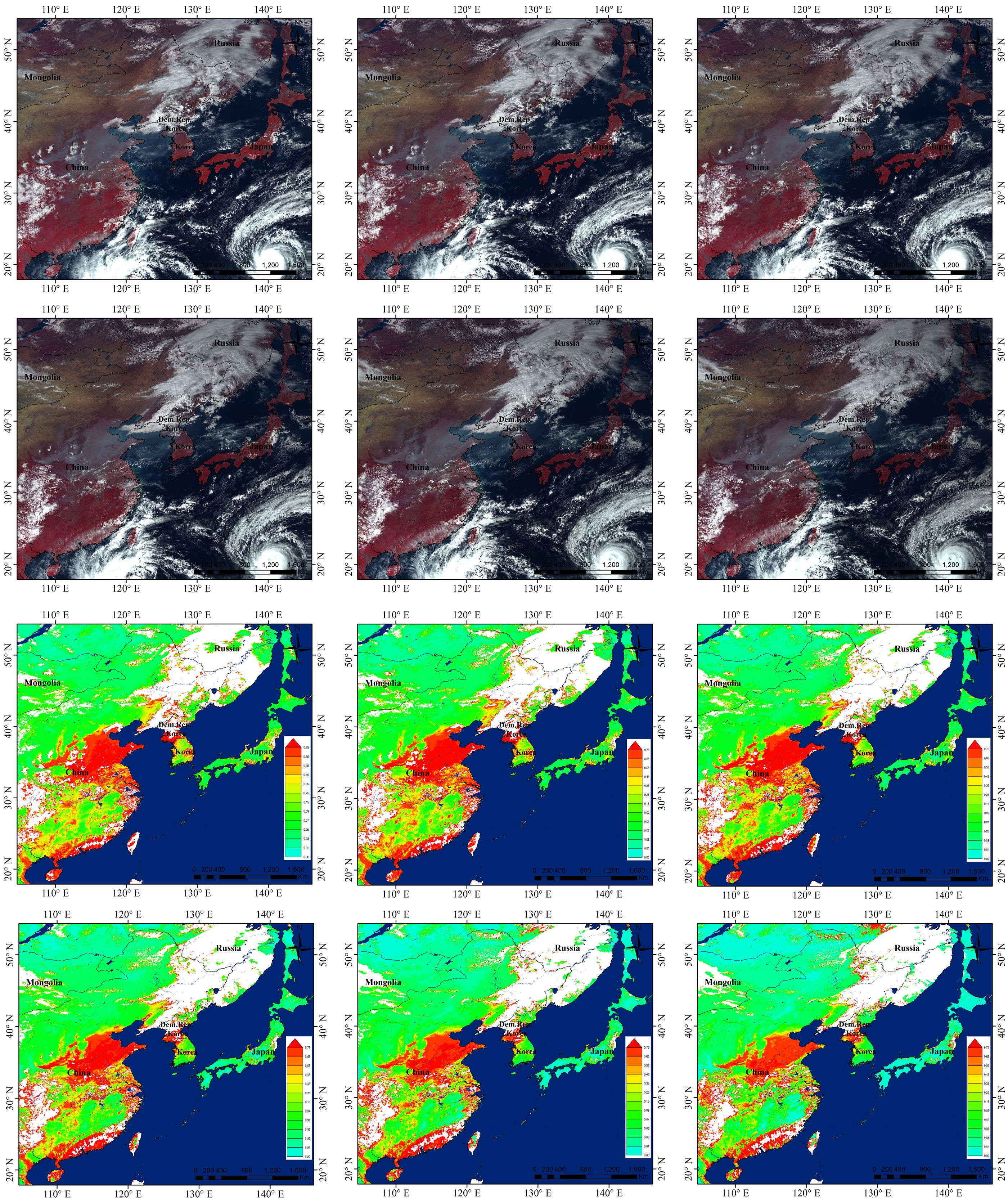The color photograph displays a 4x3 grid comprising 12 images, presenting detailed views of weather patterns over various land masses and oceans. The top six images, resembling satellite photographs, highlight cyclone-shaped clouds and white storm formations moving across regions, alongside directional markers indicating latitudinal and longitudinal coordinates (e.g., 50°N to 20°N, 110°E to 140°E). This section emphasizes real-time weather systems, possibly hurricanes, and their impact on different continents, with vivid splashes of red, black, brown, and swirling white clouds against the dark ocean. The bottom six images transform into heat maps, depicting temperature fluctuations using a spectrum of colors—from green to red—showing the severity of the storms and temperature variations on land. These heat maps are accompanied by a legend that deciphers the color codes, enhancing the depiction of hotter and cooler areas. The vibrant visuals, with shades of green, red, white, yellow, and blue, make a stark contrast to the top-view images, offering a comprehensive understanding of weather conditions over the specified regions.